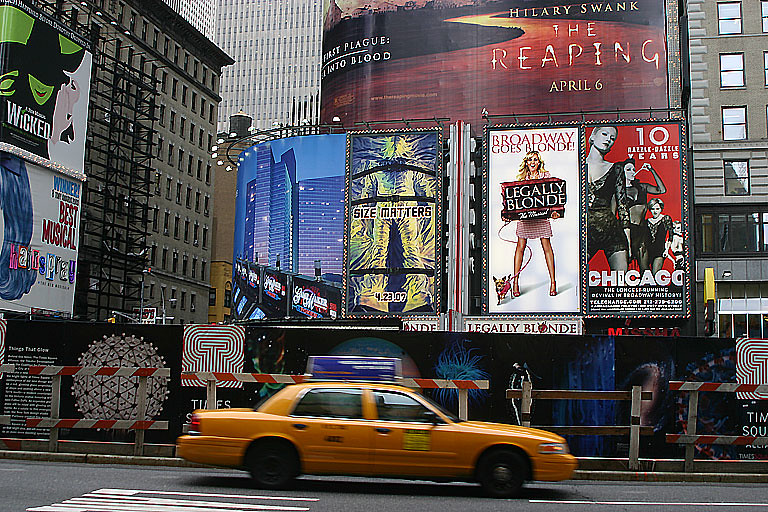The image features a bustling city street dominated by a yellow taxi in the bottom center. The taxi has a blue sign on its roof and a yellow sign on its passenger door, with black wheels adding contrast. Behind the taxi, the background is rich with various posters and signs, including roadblock equipment placed on the sidewalk. 

The prominent posters and billboards around the street enhance the urban atmosphere. There's a large billboard on top of a building that announces "Hillary Swank, The Reaping, April 6th." Nearby, another poster promotes "Legally Blonde" the Broadway show, and further to the right is another sign for the show "Chicago," marked with the number "10." On the building to the left, which has multiple small windows, there is a notable billboard with a green-faced witch wearing a black hat that says "Wicked," below which is another blue sign. Additionally, behind the taxi is a wall painted with a maze.

To the right of this building, another shorter, seven to eight-story building stands tall, adorned with its own set of billboards. Some of the signs suggest ongoing construction, as indicated by the red and white striped fences. Furthermore, visible signs also advertise "Size Matters" and proclaim "Best Musical" in red letters against a backdrop of black and white graphics. The combination of these visual elements captures the vibrant and dynamic essence of city life.